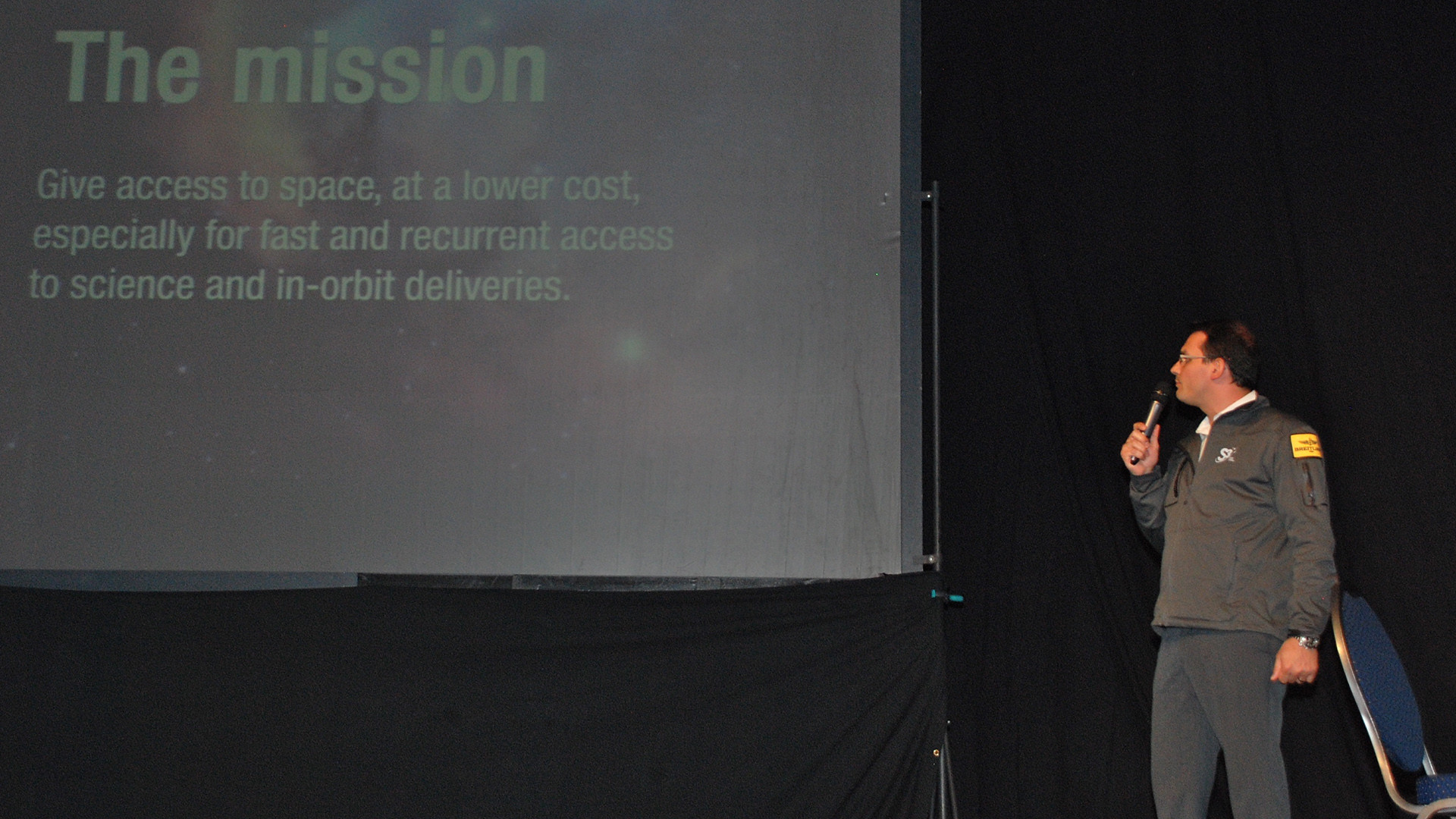In this picture, a man is giving a presentation, standing in front of a projector screen that features a night sky background adorned with galaxies and stars. The projected text reads: "The mission: give access to space at a lower cost, especially for fast and recurrent access to science and in-orbit deliveries." 

The man, positioned to the right of the screen, has black hair and is wearing glasses. He is dressed in a black windbreaker jacket with a yellow sticker on the side, a white shirt underneath, and black trousers. His right hand holds a microphone, indicating he is speaking to an audience. Behind him, there is a blue chair oriented to the right side of the picture. The primary colors in the image are black, with touches of green in the text and blue in the chair.